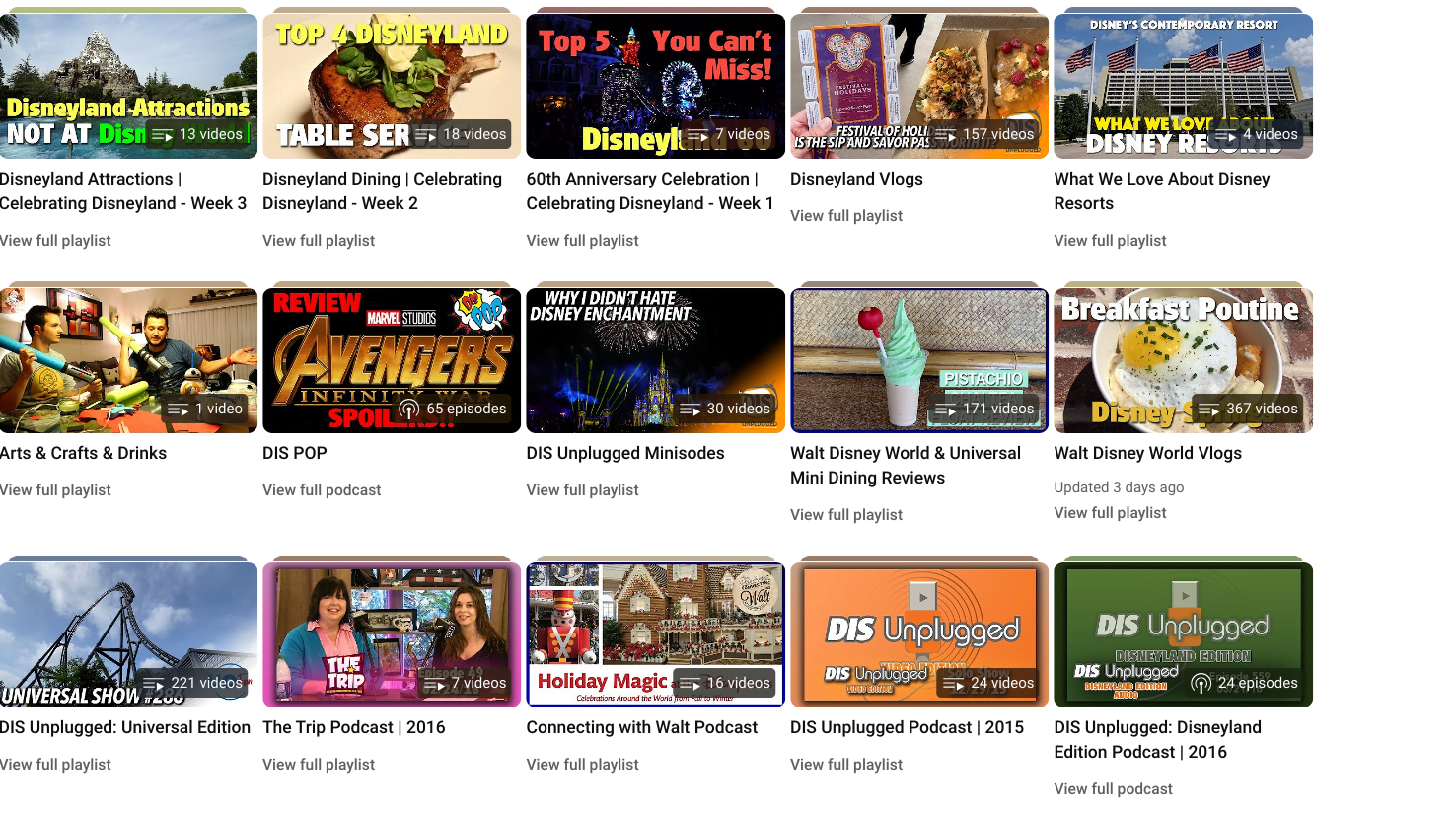A detailed screenshot showcasing a YouTube-like interface with a variety of video thumbnails organized in rows. Each thumbnail features a distinct image, highlighting different aspects of Disney experiences.

In the top row, the thumbnails emphasize various Disneyland and Disney World attractions and reviews:
1. "Disneyland Attractions" - Shows a collage of popular attractions.
2. "Top Four Disneyland Table Service" - Focuses on dining options.
3. "Top Five Can't Miss Disneyland" - Lists essential experiences.
4. "Disneyland Vlogs" - Highlights personal vlog content.
5. "What We Love About Disney Resorts" - Features resort highlights.

The second row continues with Disney-related content:
1. "Arts and Crafts" - Displays creative Disney-themed projects.
2. "Drinks" - Shows two men with lightsabers, indicating themed beverages.
3. "Disney Pop" - Offers a review of an Avengers movie.
4. "Why I Didn't Hate Disney Enchantment" - A review on the Disney Enchantment show.
5. "Walt Disney World and Universal Mini Dining Reviews" - Showcases dining options at both parks.
6. "Walt Disney World Vlogs" - Personal vlogs about Disney World experiences.
7. "Breakfast Poutine" - A unique Disney dining option.

The bottom row predominantly features Disney-themed shows and podcasts:
1. "Universal Show" - Everything related to Universal Studios.
2. "Dis Unplugged Universal Edition" - A podcast devoted to Universal Studios.
3. "The Trip Podcast 2016" - A travel podcast episode from 2016.
4. "Connecting with Walt Podcast" - Focuses on the legacy of Walt Disney.
5. "Some Holiday Magic" - Showcases Disney holiday events.
6. "Dis Unplugged Podcast 2015" - A 2015 podcast episode.
7. "Dis Unplugged Disneyland Edition Podcast 2016" - A 2016 Disneyland-focused podcast episode.

Each thumbnail represents a collection of videos, inviting viewers to explore multiple pieces of content within each category.